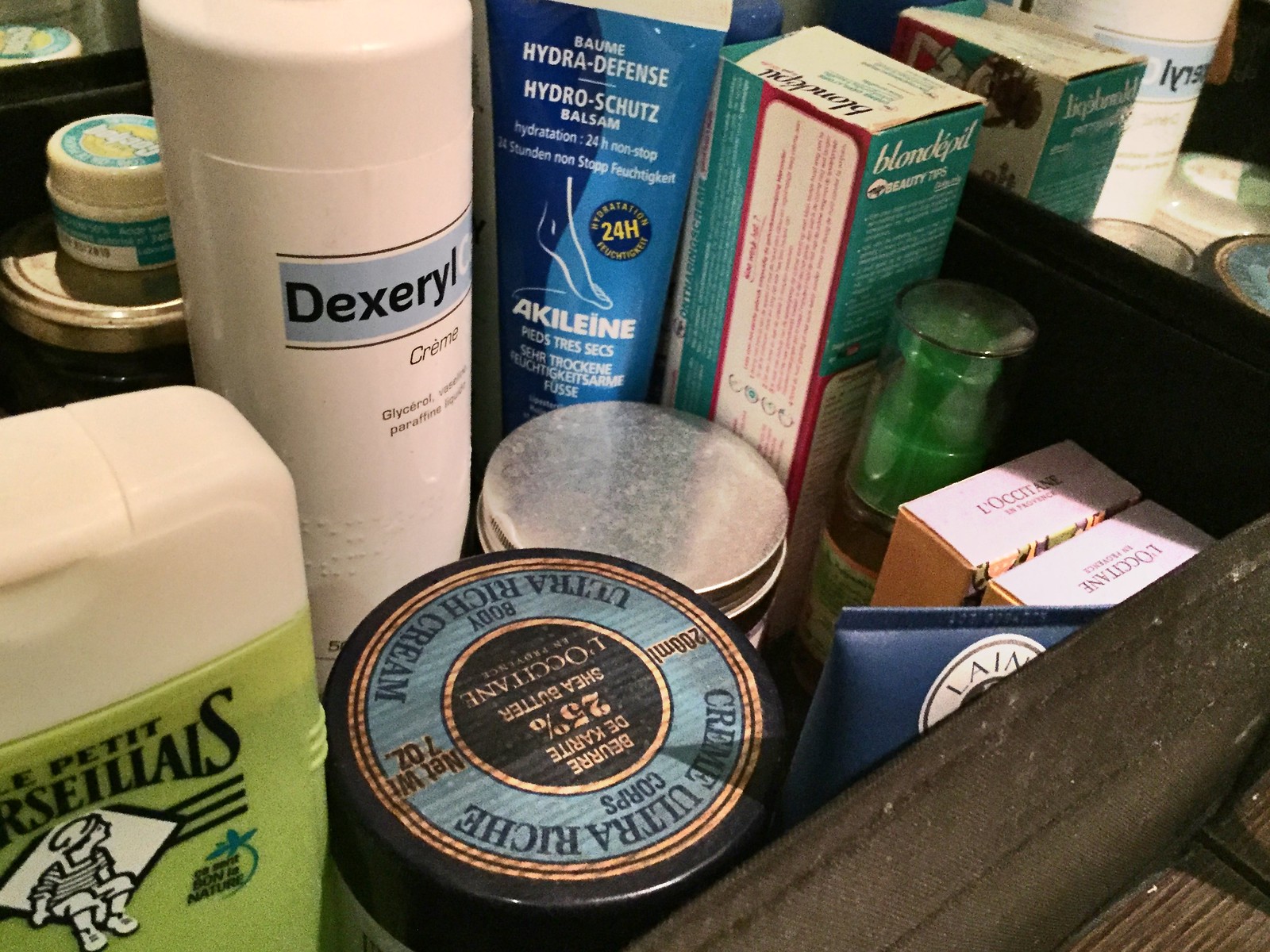A meticulously arranged collection of beauty products is showcased on a rustic brown wooden shelf or crate, which rests on a similarly colored wooden green-hued countertop. Adjacent to the display stands a mirror, reflecting the scene. The display features an assortment of 10 or 11 diverse beauty items.

Starting from the far left, a mysterious green-hued beauty product commands attention, its purpose not immediately clear. Next in line is an ultra-rich cream housed in a tub with a black lid, labeled "Cream Ultra-Rich." Following the rich cream, a blue squeezy tube sits, its label obscured from view.

Two adjacent closed boxes are labeled "Locte," their exact nature unconfirmed. They are followed by a serum, visibly identifiable by its lid, leading to an unidentifiable tub crowned with a silver lid. Nearby, a box that might contain toothpaste holds its place in the arrangement. 

Further along, a blue squeezy tube marked as some type of hydro-defense foot cream stands out. Beside it, a white container is labeled "Dexeral" with additional text that remains unclear. Rounding out the lineup is another type of cream, and positioned on a higher shelf behind the primary display is a small, unidentifiable tub.

The variety and arrangement of these beauty products create a visually appealing and detailed still life, inviting curiosity about the specifics of each item.